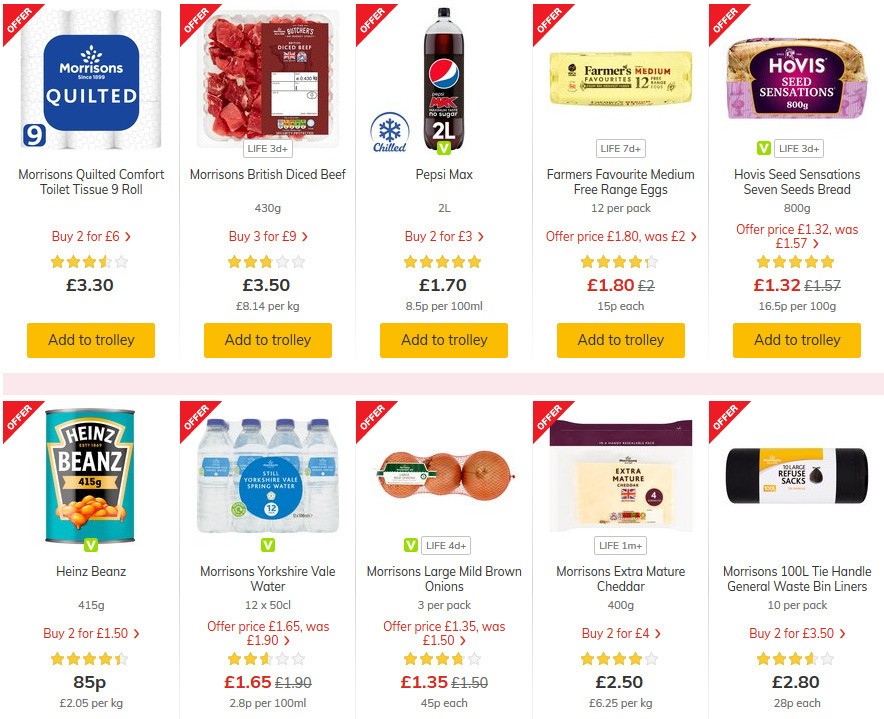In this image, a detailed list of various grocery items is presented on a page, containing a total of ten different products. The first item is Morrison's Quilted Comfort Toilet Tissue, available in a nine-roll pack. The second item on the list is Morrison's British Diced Beef. Next, we have a listing for Pepsi Max. The fourth product is Farmer's Favourite Medium Free-Range Eggs. Following that is Harvest Seed Sensations 7-Seeds Bread. Skipping to the seventh item, we find Heinz Beans. The eighth product is Morrison's Yorkshire Veal Water. Also listed as the eighth item, there is Morrison's Large Marbled Brown Onions. The ninth product is Morrison's Extra-Mature Cheddar. Finally, the tenth item is Morrison's 100-Liter Thai Handle General Waste Bin Liners.